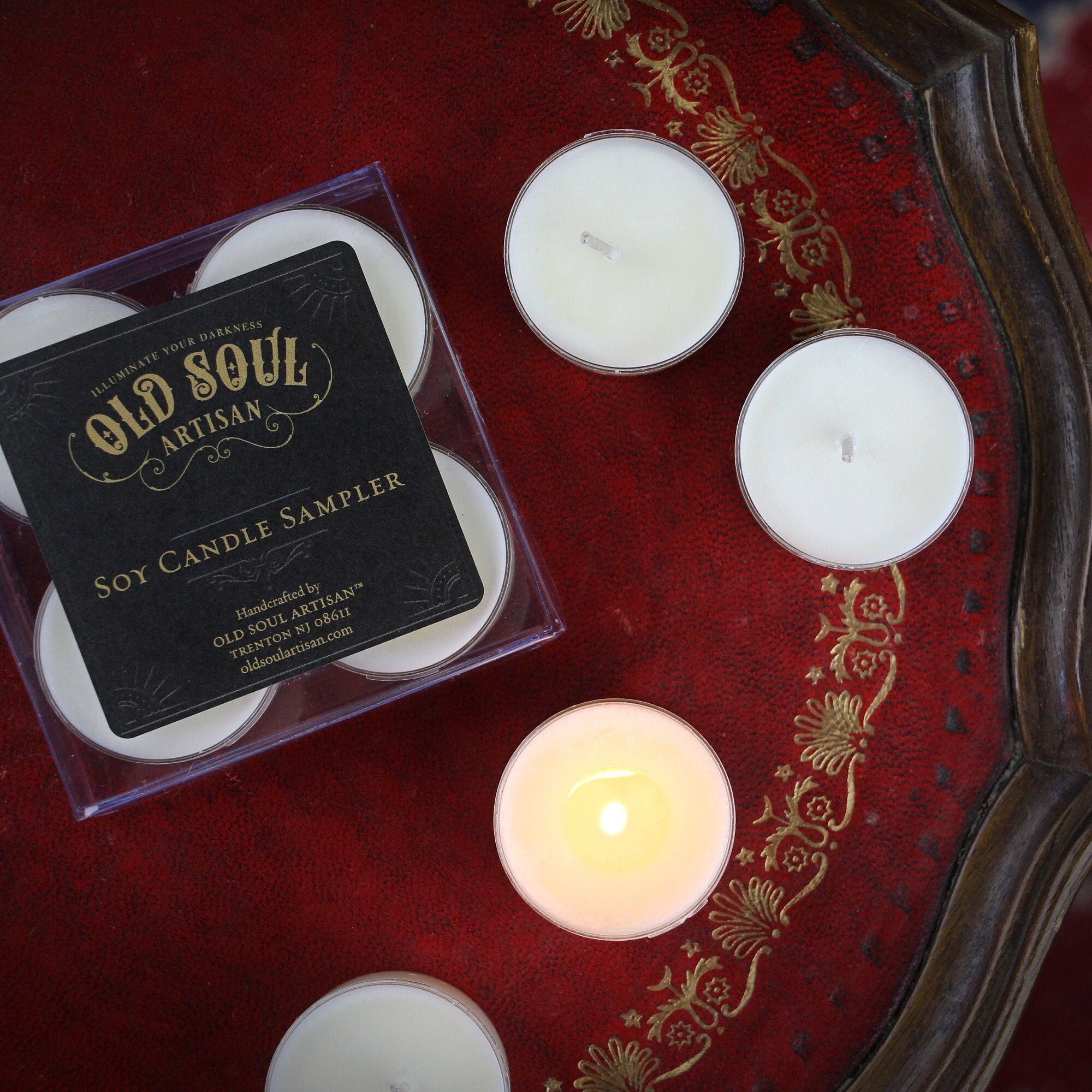The image captures an indoor scene featuring a burgundy-red velvet table adorned with an ornate wooden edge and gold trimming. The table, set against a maroon carpet backdrop, displays a collection of small, white tea light candles in short glass jars. Four candles sit freely on the table, while another four are encased in a clear plastic box labeled "Old Soul Artisan Soy Candle Sampler." The label also includes additional details: "Illuminate Your Darkness," "Handcrafted by Old Soul Artisan, Trenton, New Jersey 08611," and the website "oldsoulartisan.com." The meticulously arranged candles, both boxed and unboxed, add a touch of elegance to the setting, though none are lit.